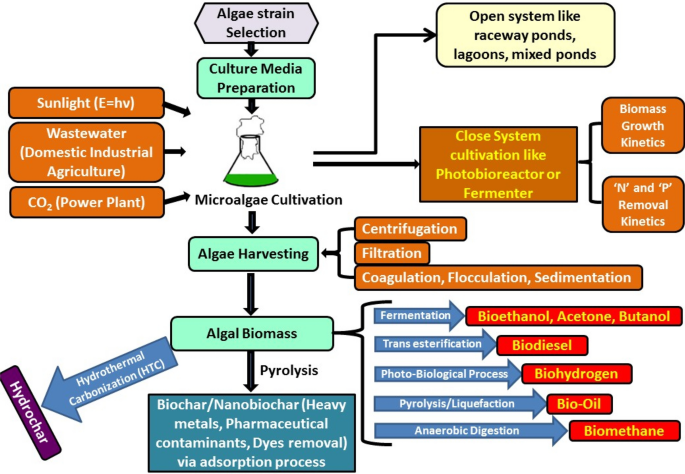This detailed horizontal flowchart illustrates the comprehensive process of algae cultivation and water reprocessing, with a focus on scientific methodology and treatment steps. It begins with "algae strain selection" at the top, followed by "culture and media preparation." A central flask filled with green algal media and foam is depicted, with several arrows directing the flow of processes.

To the left of the flask, three boxes indicate essential inputs: "sunlight (E=hv)," "wastewater (domestic, industrial, agricultural)," and "CO2 (power plant)." Below the flask, the steps "microalgae cultivation" and "algae harvesting" are outlined, leading to "algal biomass."

From the flask, arrows branch out to various cultivation systems: "open systems like raceway ponds, lagoons, mixed ponds," and "closed system cultivation like photobioreactors or fermentors." Adjacent to these, it describes "biomass growth kinetics" and "N and P removal kinetics."

To the right of the algae harvesting box, methods such as "centrifugation," "filtration," "coagulation," "flocculation," and "sedimentation" are shown for processing. Further steps include "hydrothermal carbonization (HTC)" leading to "hydrochar" and "pyrolysis," resulting in "biochar," "nanobiochar," and specifying applications like "heavy metals, pharmaceutical contaminants, dyes removal via absorption process."

A set of five blue arrows stemming from "algal biomass" highlight downstream processes: "fermentation," "transesterification," "photobiological process," "pyrolysis and liquefaction," and "anaerobic digestion." These processes yield various bio-products illustrated in red boxes: "bioethanol, acetone, and butanol," "biodiesel," "biohydrogen," "bio-oil," and "biomethane." The illustration employs a mix of orange, green, and dark blue boxes with black and white text, complemented by yellow and white lettering, and black arrows guiding the entire flow.